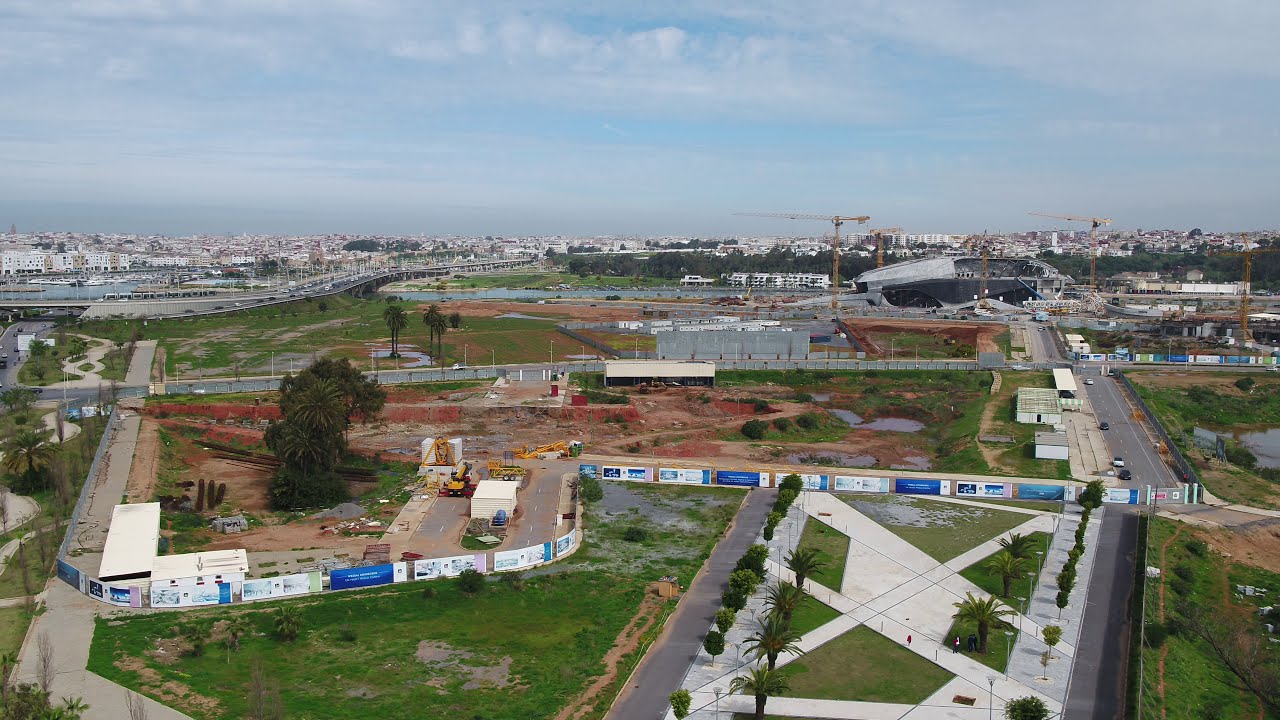This overhead photograph captures a dynamic, sprawling cityscape characterized by a bustling mix of completed and under-construction areas. The upper third of the image is dominated by a cloudy sky with hints of blue peeking through, creating a somber backdrop for the scene below. In the distance, a densely packed urban area features numerous buildings, while several tall cranes punctuate the skyline, indicating ongoing construction.

In the foreground, the photo reveals a construction site surrounded by a jagged fence lined with blue and white advertisements. This fenced-off area includes overturned dirt, mounds, and scattered puddles, giving the impression of recent activity or rainfall. Adjacent to the construction zone, on the bottom right, lies a more developed section with diagonal concrete sidewalks, landscaped with palm trees, suggesting a tropical climate.

Winding roads snake vertically and horizontally through the frame, densely populated with vehicles, underscoring the area's high level of traffic. Scattered across the scene are various plots of land, some fenced off, with a blend of unkempt grass and landscaped spaces.

To the right, a park-like area with walkways cuts a more orderly contrast to the chaotic construction, featuring numerous palm trees. The photo appears to be taken from a high vantage point, offering a comprehensive view of this vibrant, urban landscape, encapsulating the juxtaposition of development and nature interwoven throughout the scene.